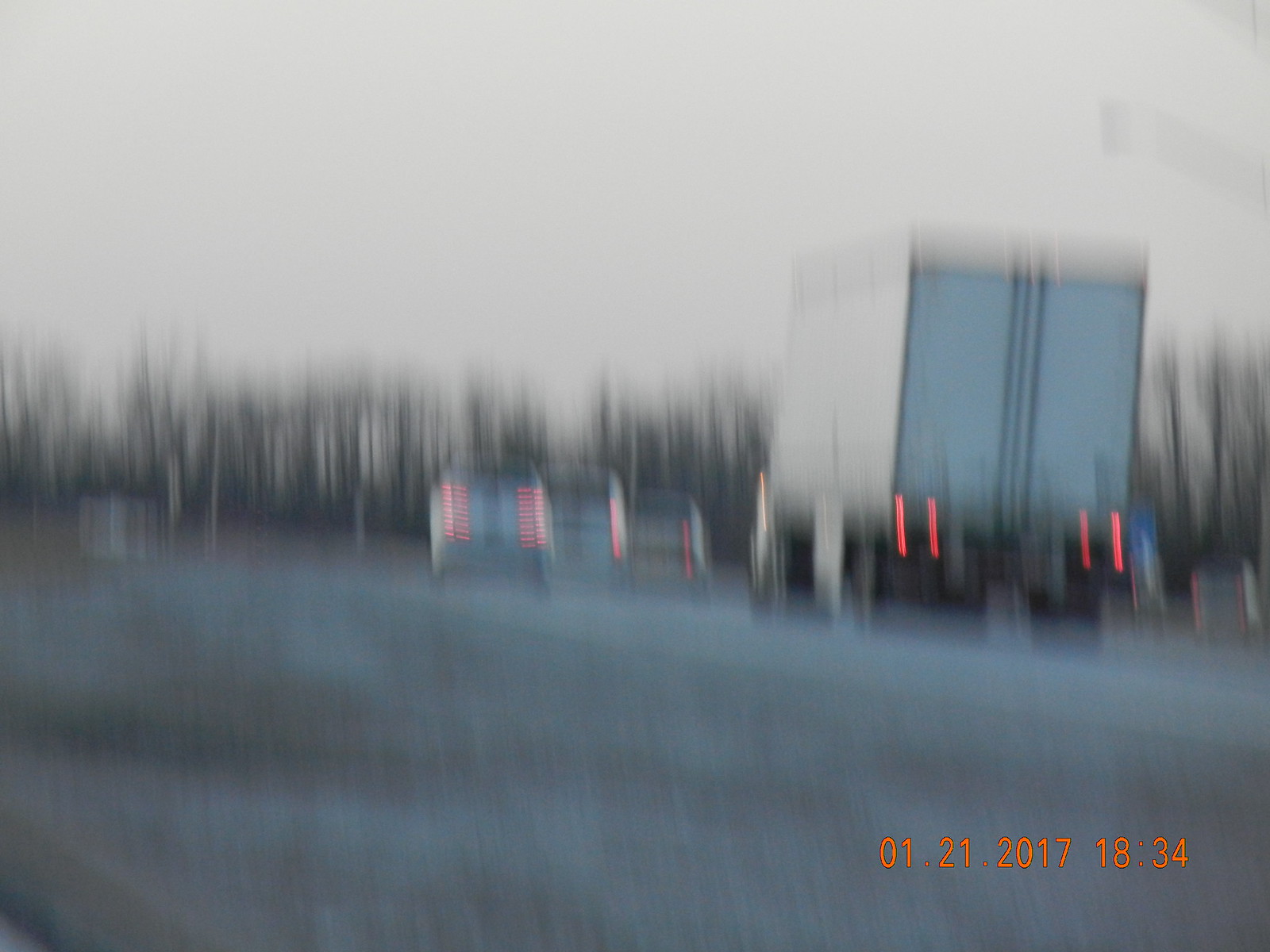Captured on January 21, 2017, at approximately 6:34 PM, this photograph, likely taken with an old-school film camera, exudes a nostalgic yet somber tone. The image features a road spanning the bottom portion, with several vehicles gathered in the bottom right corner, all displaying their brake lights. Dominating the foreground is a white truck, its brake lights glowing red. To its left, another car has also engaged its brake lights, followed by two more vehicles ahead, similarly illuminated. The scene is enveloped in a muted, monochromatic palette, under a cloudy winter sky. Bare trees, devoid of leaves, stand starkly in the background, further enhancing the photo's wintry, gray ambiance.